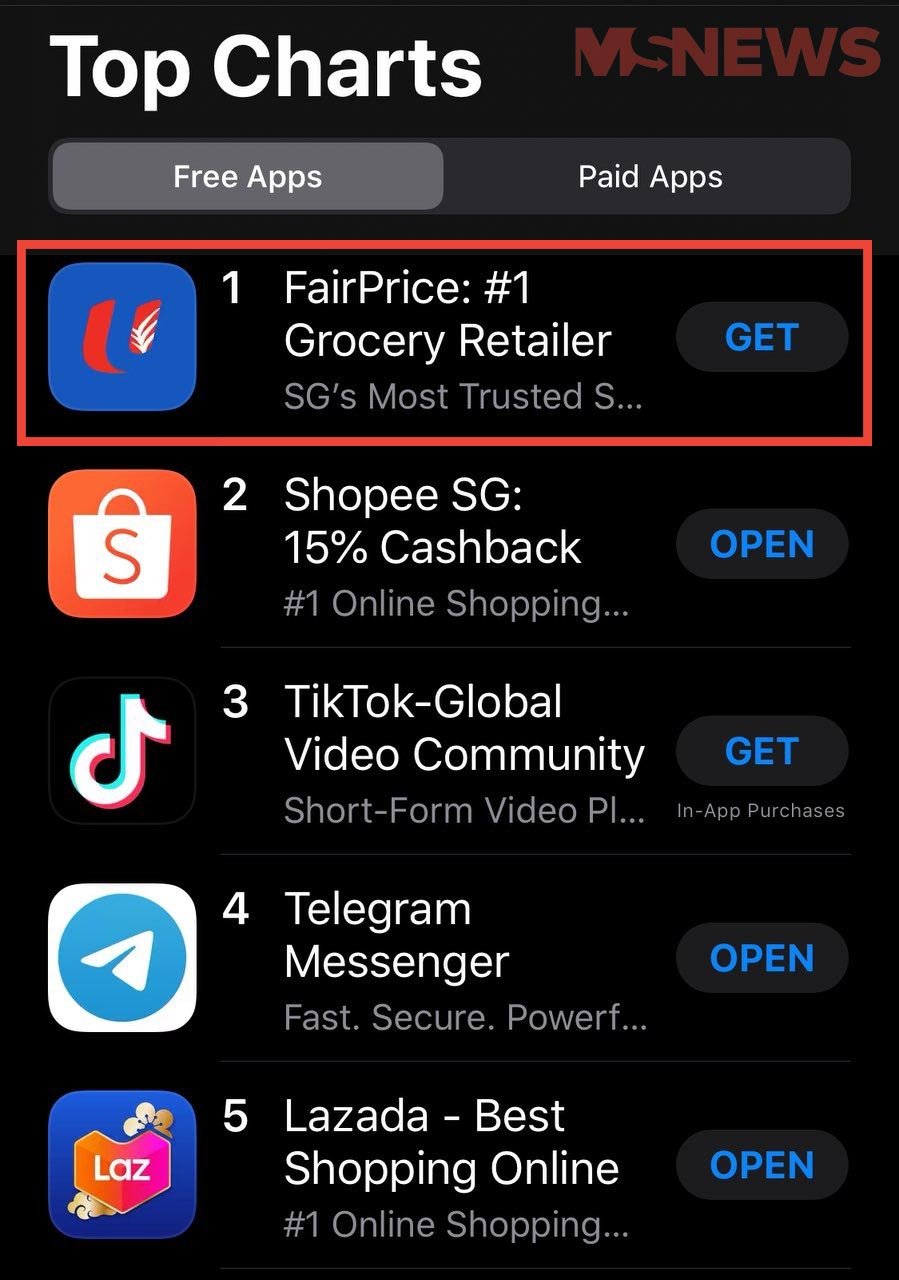The image showcases a screenshot from a tablet, featuring a chart of top apps set against a solid black background. At the upper left corner, the bold white text reads "Top Charts." On the upper right, the logo for "MS News" is displayed in red text, except for the letter "S," which is in black.

Below the header, there are two buttons: on the left, a grey button labeled "Free Apps," and on the right, a button labeled "Paid Apps."

The main section of the screenshot highlights the top-ranked apps, each listed within a red outline. The first app is "FairPrice No. 1 Grocery Retailer," which features a blue icon resembling a feather on the left side and a "GET" button on the right. 

The second app, "ShopeeSG," is accompanied by the text "15% Cash Back, No. 1 Online Shopping," and an "OPEN" button to the right.

In the third position is "TikTok Global Video Community," with a "GET" button to the right.

Following TikTok, the fourth app listed is "Telegram Messenger," and lastly, in the fifth position, is "Lazada," described as "Best Shopping Online."